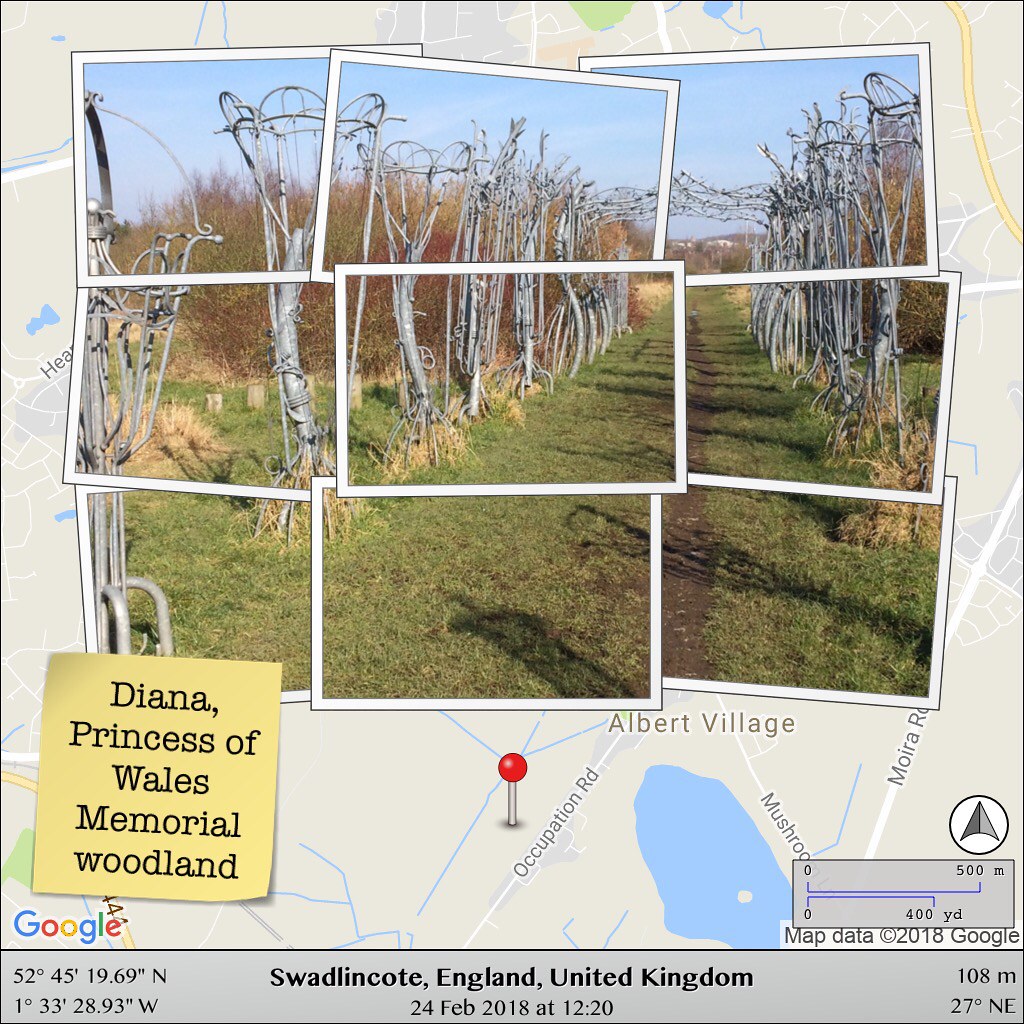The image is a composite consisting of a Google Maps background with an overlay of nine individual photographs arranged to form a cohesive view of a location. The background map, recognizable by the Google logo and map data copyright 2018 Google text, features a pin marking the Diana Princess of Wales Memorial Woodland. The foreground images depict a scenic grass area flanked by newly planted trees and taller grasses, all framed to resemble a stack of photos with white borders placed at angles. A yellow rectangle in the lower left corner serves as a makeshift sticky note, reading "Diana Princess of Wales Memorial Woodland." At the very bottom of the image, across a gray bar, it is labeled "Swadlincote, England, United Kingdom, 24th February 2018 at 12:20." This detailed overlay offers a visually engaging representation of the memorial woodland's location and its environment.